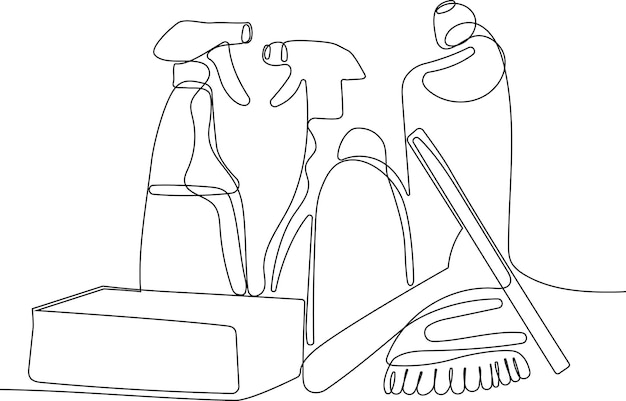This is a black and white continuous line drawing that depicts various cleaning supplies. The fine line, which appears to have never been picked up, intricately wraps around and creates the three-dimensional forms of the objects. In the foreground, there's a sponge, a squeegee, and a brush with a handle. In the background, four bottles are arranged—two spray bottles and two squirt bottles, one with a twisted neck suggesting it might be for toilet bowl cleaner, and you can see fluid in one of the bottles on the left. Despite some elements not being fully closed, the abstract, AI-generated style effectively captures the essence and dimensions of the cleaning tools set against a simple white background.